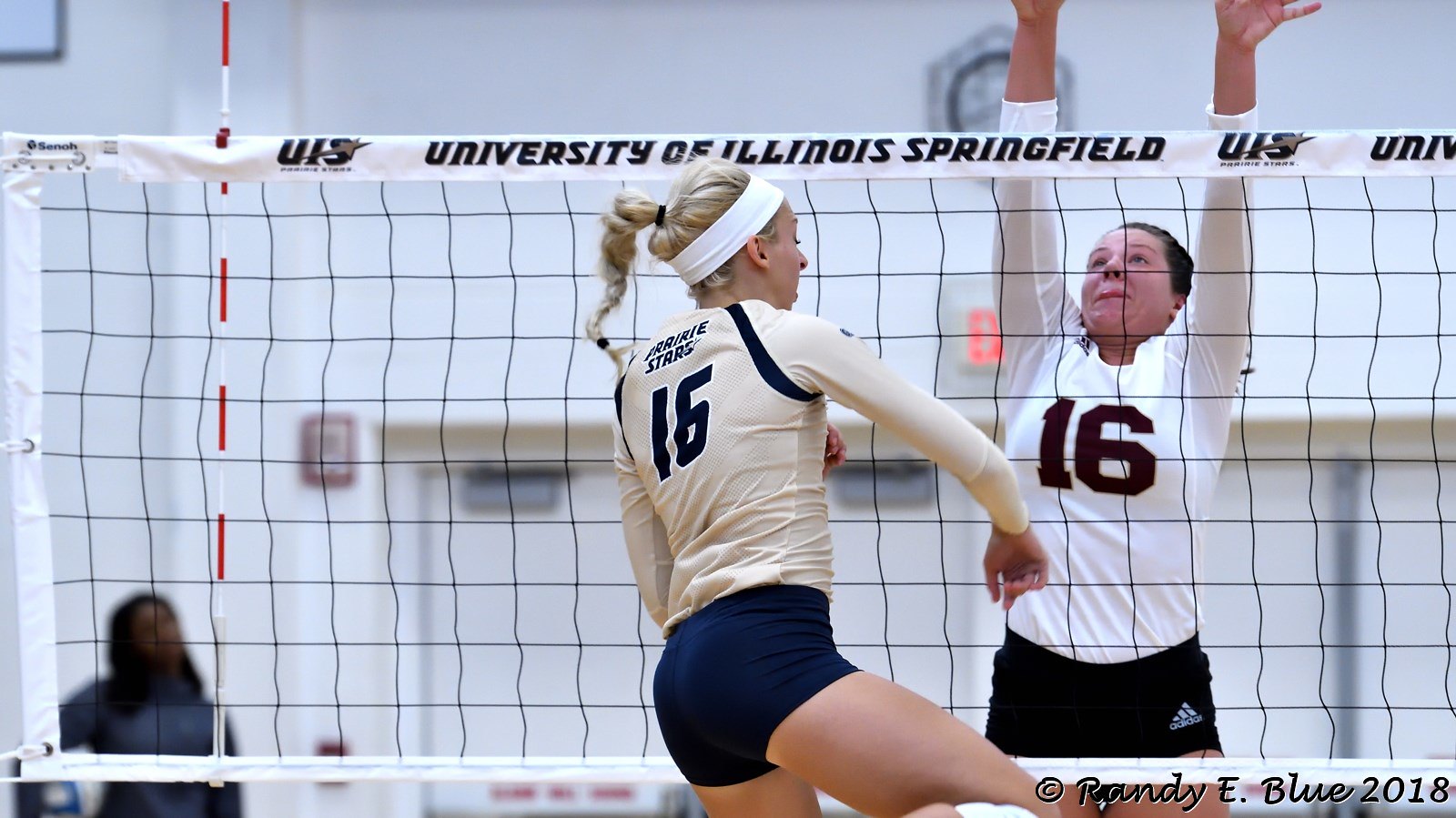In this color photograph capturing the intensity of an indoor volleyball match, two women are prominently featured at the net. The foreground showcases a player in motion, just having completed a hit. She is facing away from the viewer, dressed in a tan-colored jersey with the blue number 16 on the back, paired with blue shorts and a white headband. Her blonde hair is pulled back in a ponytail, allowing her focus and determination to shine through. Opposite her, across the net, stands her opponent, facing the viewer with arms outstretched, ready to block the spike. This player is clad in a white jersey, also emblazoned with the number 16 in black, and black Adidas shorts. The fully extended net spans the image's width, marked by a white strip at the top and bottom, with "University of Illinois Springfield" boldly inscribed along with its logo. The photograph’s realistic detail captures not only the players' dynamic actions but also the environment, with a blurred spectator in the background, ensuring the viewer’s attention remains on the athleticism and competitive spirit of the moment. The image is credited to Randy E. Blue, 2018, a hallmark of photographic representationalism realism.